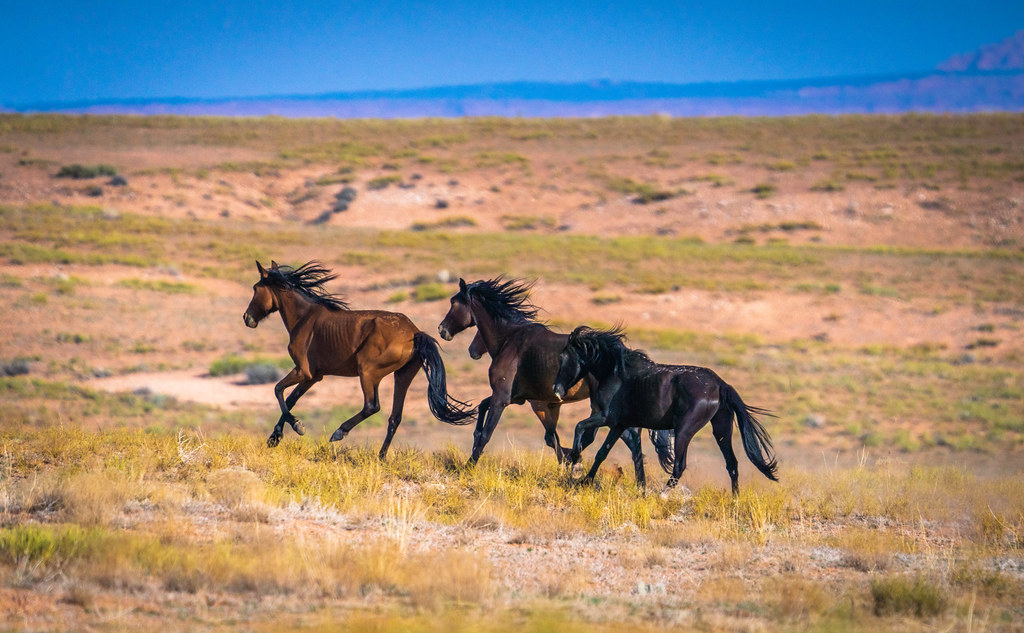In this vivid and striking landscape photograph, three wild horses race through an open, sun-drenched field. The terrain appears mostly arid, with sparse patches of grass, weeds, and small plants scattered among rocks and dirt. In the distance, gentle hills can be seen under a bright blue sky that subtly transitions into shades of purple, enhancing the midday's warmth. The horses, unburdened by any saddles, are captured in mid-gallop, aligned in a staggered formation with their powerful black manes and distinctive black legs clearly visible. Leading the trio is a light honey-brown horse, followed by a chocolate brown horse, and lastly, a dark brown or near-black horse. Each horse runs free, embodying the spirit of the untamed wilderness.